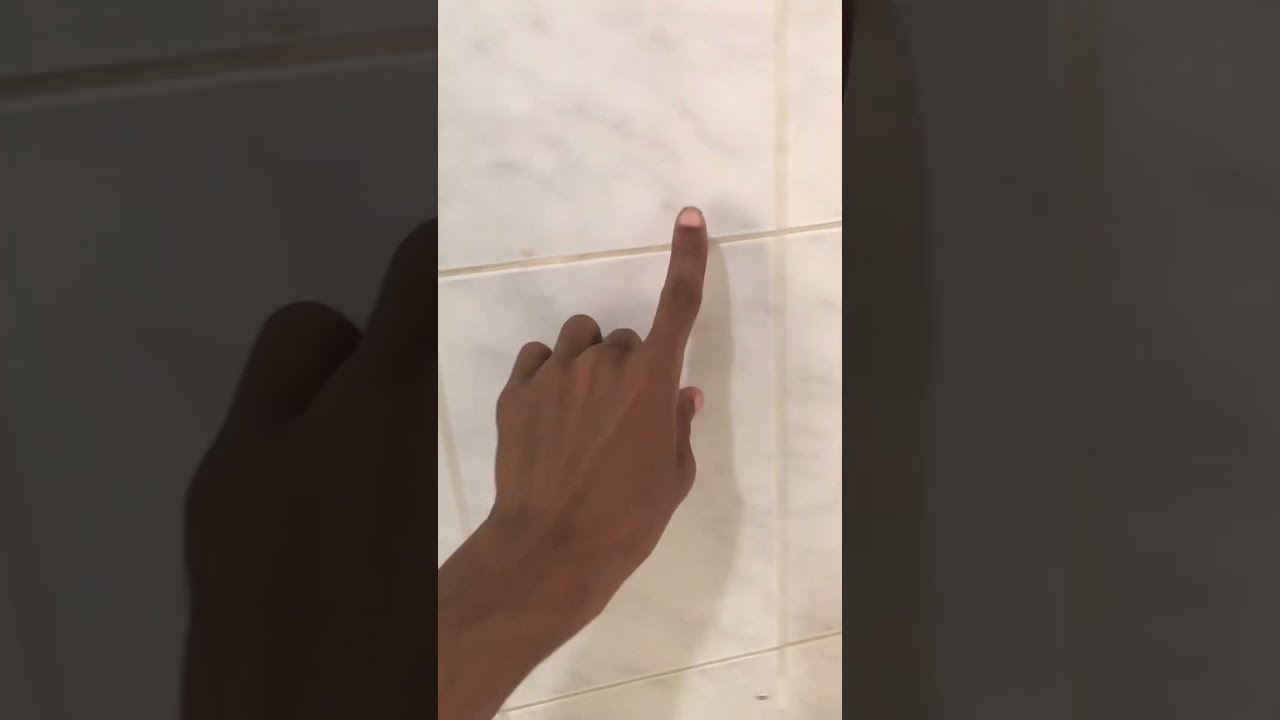In this detailed image, a dark-skinned hand with the index finger pointing up is prominently displayed against a backdrop of large, square, white marble tiles with delicate gray veining. The hand, likely that of an Indian man, extends from the bottom left towards the center of the image. The other fingers are bent, and subtle veins are visible on the back of the hand. The thumbnail appears polished in a light pink color. The tiles have a light cream-colored grout, which looks a bit worn and dirty in spots. The main image is well-lit with good indoor lighting, casting a clear shadow of the hand on the tile. Flanking the central image are grayed-out, zoomed-in sections of the same scene, highlighting just portions of the hand and the tile. These sections are darker compared to the well-lit center, with noticeable shadows and marbling swirls on either side. The entire scene suggests the setting is likely a bathroom, with the pristine yet subtly aged appearance of the tiles enhancing the overall composition.